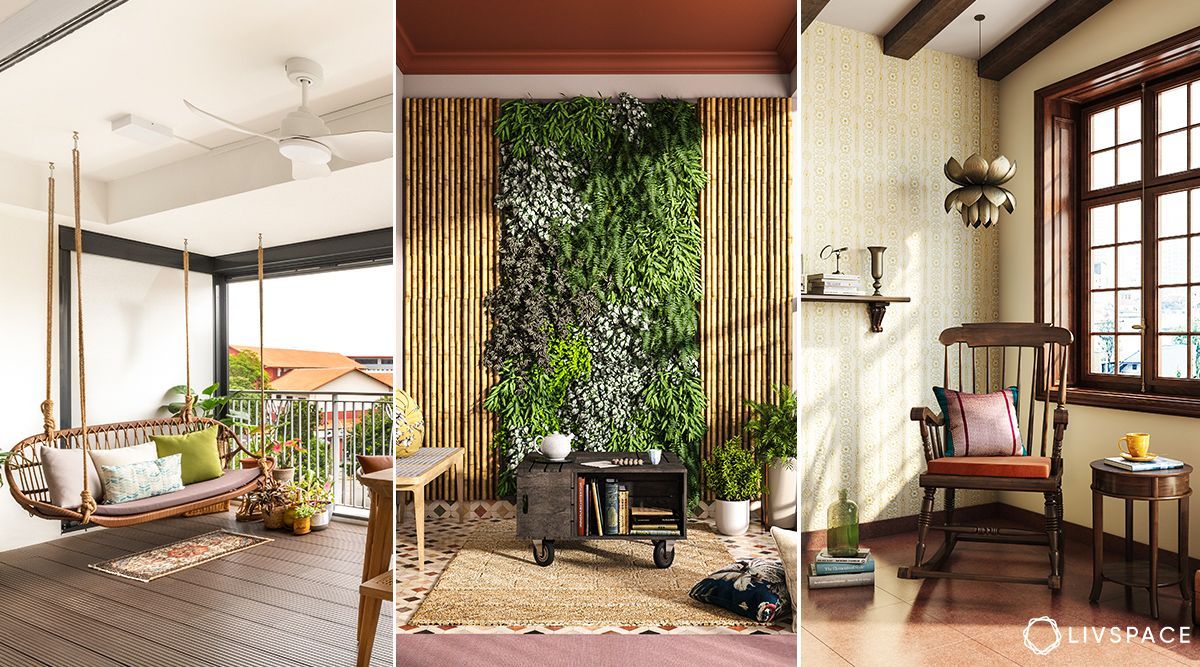This is a detailed collage of three indoor scenes, each depicting a cozy and inviting setting.

On the left side, the image showcases a hanging swing chair suspended from the ceiling with ropes. The swing is adorned with four fluffy pillows—one green and three light-colored—resting on a rug. This room features white walls and a wooden floor, with a ceiling fan above. The space opens up to a patio through a sliding door, revealing outdoor views, likely of neighboring rooftops. Several plants add a touch of greenery to the setting, enhancing its inviting atmosphere.

The middle image presents a room that appears to be a reading or relaxation nook. The focal point is a wall adorned with lush houseplants, creating a vertical garden effect. At the base of this green wall sits a small desk or table topped with a potted plant. A carpet covers most of the wooden floor, and additional potted plants are visible around the room. The ceiling is brown, complementing the natural, earthy feel of the space.

On the right side, the image features another room centered around a brown rocking chair. Near the chair, a small table holds a cup and saucer and a book. On the floor beside it, there are a couple of books stacked with a glass bottle atop them. The room features a wooden floor, white walls, and a window with a brown frame that lets in natural light. A lamp with a bottle-shaped base adds a unique decorative touch. Behind the rocking chair, there is a shelf providing additional storage and decorative options.

Each image collectively highlights a blend of rustic and modern elements designed for comfort and relaxation, making it an appealing advertisement for a home or a short-term rental property like Airbnb or VRBO.